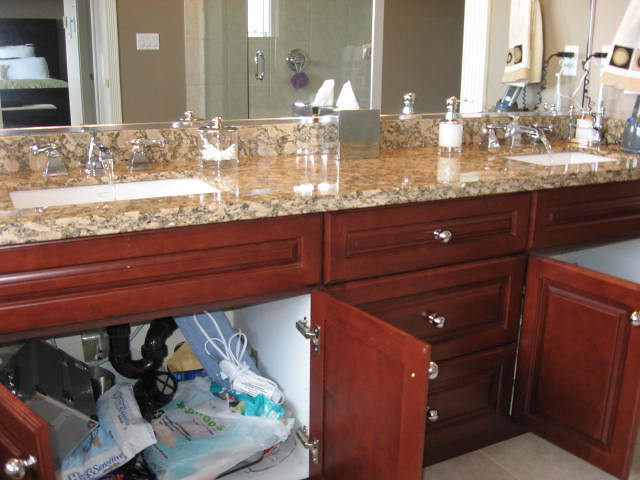This photograph captures a well-appointed bathroom countertop featuring two matching sinks embedded in a luxurious stone or synthetic surface designed to mimic marble. The countertop showcases an intricate pattern of grayish-brown veins set against a backdrop of ecru or light beige. Each sink is accompanied by a set of two-handled faucets, each with a single spout. Centrally located between the sinks, a tissue dispenser is neatly placed, flanked by elegant pump soap dispensers with white bodies and silver tops.

Above the countertop, a large mirror reflects a fragment of the shower area, including the door and its handle. In the upper left corner of the image, an open section of a cupboard is visible, stocked with neatly arranged towels. Meanwhile, in the upper right corner, an electric outlet is occupied by plugged-in devices with dangling cords, and a towel hangs from a rack nearby.

Dominating the lower portion of the image, the dark wood-stained drawers and cupboards display a balance of functionality and design, with shiny round handles adding a touch of elegance. However, the doors on both the right and left sides of the cupboard stand ajar, revealing a somewhat cluttered storage space beneath the countertop. Various personal care appliances, such as hair dryers and curlers, along with bags filled with miscellaneous items, are stowed haphazardly in the white-painted interior of the cupboard. The visual narrative captures a blend of meticulous style and everyday practicality.